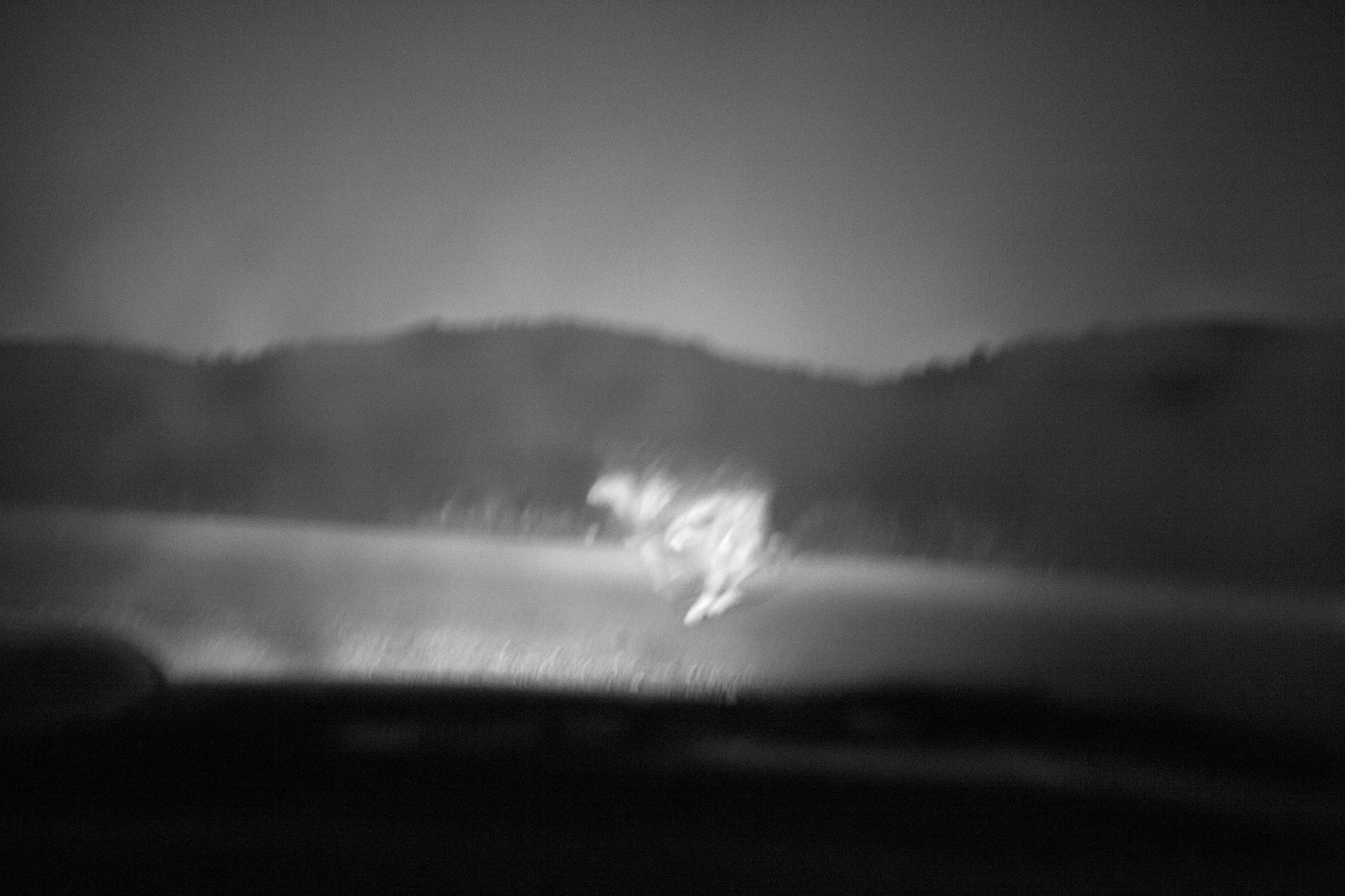This black and white landscape photograph is taken from the inside of a car, capturing the edges of the dashboard at the bottom, where the deep shadows lend a nearly black tone. Above the dashboard, a silvery gray expanse of land stretches out. It features two blurred figures, highlighted in white, whose dynamic postures suggest they might be playing soccer. The background gently rises into hills, beyond which the sky stretches, creating a muted grayscale horizon.